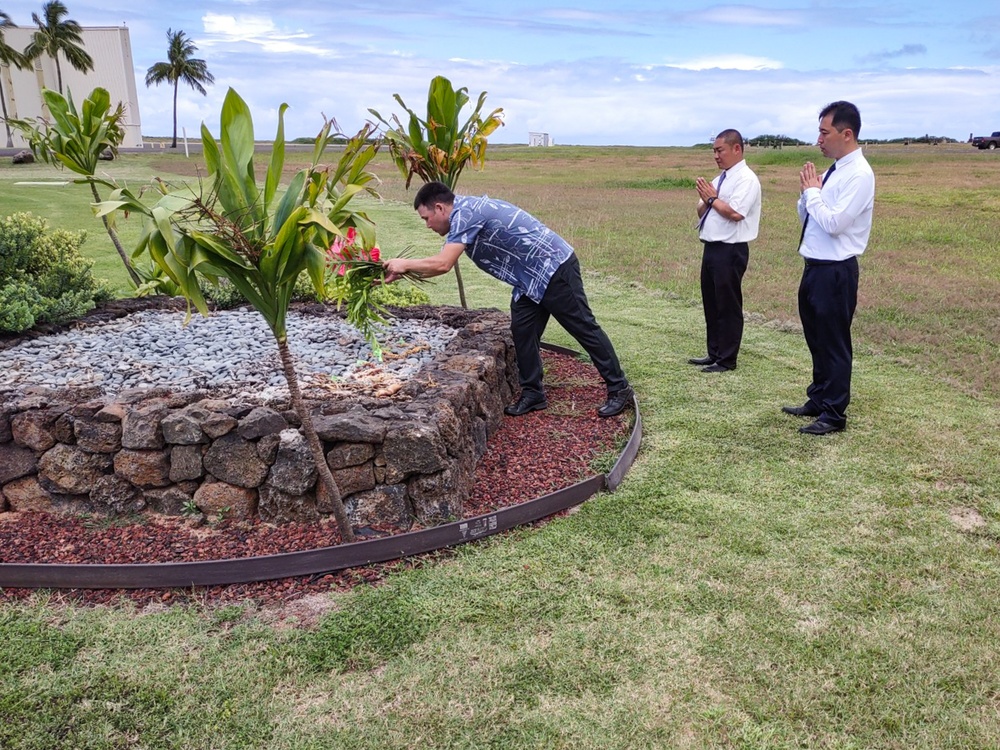The photograph captures an outdoor scene featuring three men with distinct elements repeated across the descriptions. The setting is a large open area with a grassy field occupying about 80% of the background, while the top portion reveals a blue sky with varying white and gray clouds. The focus is on a square section to the left, bordered with metal landscaping trim and filled with dark brown mulch. At the center of this section, there is a square rock structure comprising stacked dark rocks with lighter gray stones in the middle, around which tropical plants flourish.

In this landscaped area, a man wearing a blue and white patterned short-sleeved shirt, black pants, and black shoes is leaning over a green plant adorned with pink flowers. He appears to be laying a bouquet at this apparent memorial, tending to the flowers gently. Behind him stand two other men, both dressed in white collared shirts, black ties, black pants, and black shoes. They stand in the grassy field with their hands held together as though in prayer. These two men, with short black hair, direct their attention towards the man at the memorial, contributing to the solemn and reflective mood of the scene. Contrasting elements like the distant palm trees and a building in the background frame the composition, adding depth and context to the reverent moment captured in this photograph.